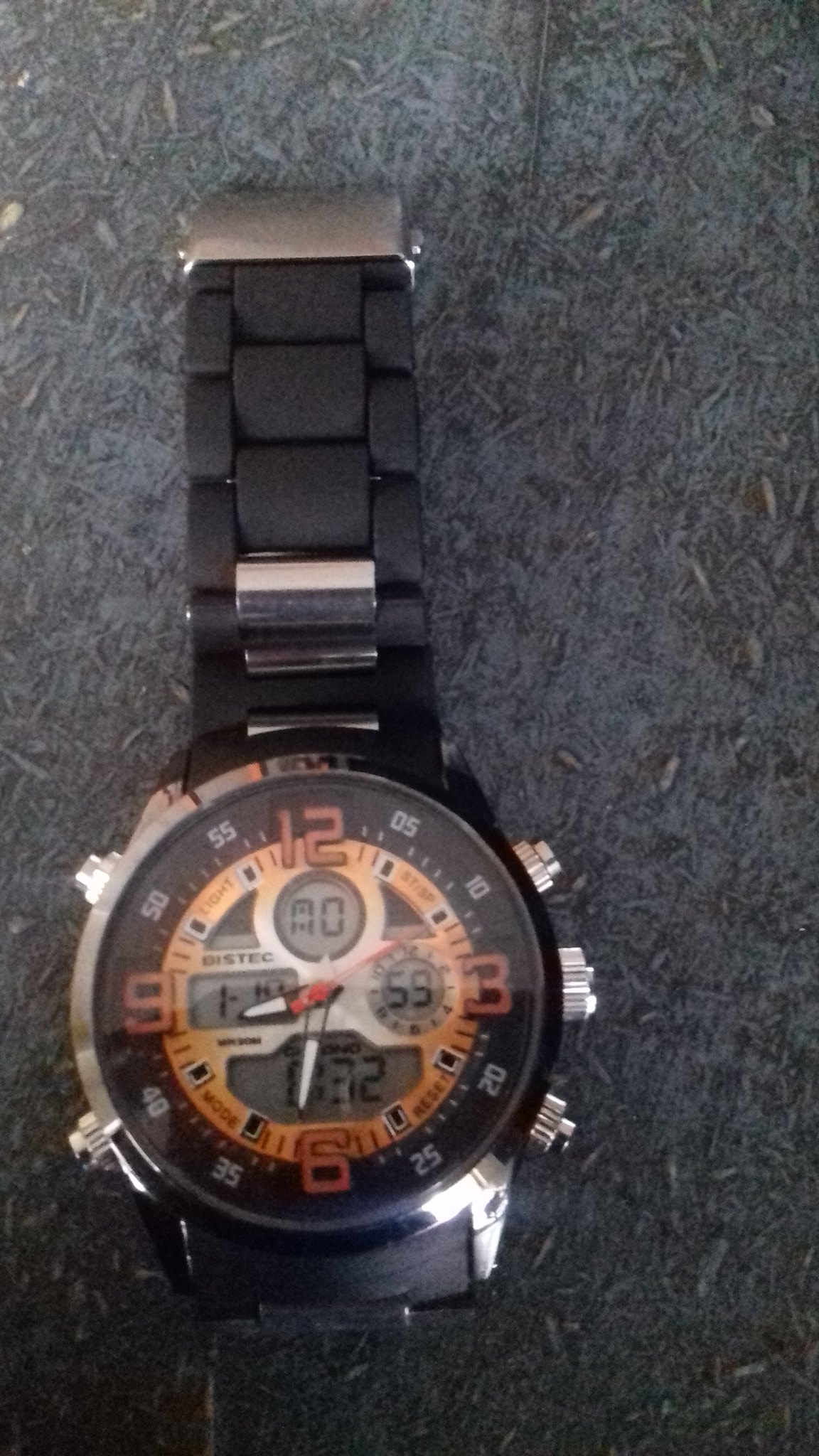This photograph features a slightly out-of-focus wristwatch lying on blue carpeting. The watch is positioned towards the bottom left of the image. It has a sleek black band, extending to the top of the frame, which includes a small metallic silver section. The main circular face of the watch, highlighted by a black and orange background, features bold orange numerals for the 12, 3, 6, and 9 o'clock positions. The rest of the design, which contains various white numbers and a digital-like display showing '0' and '59' in circular forms, adds to the watch's intricate, somewhat mechanical appearance. Additionally, silver knobs are present on both sides of the watch face, accentuating its detailed craftsmanship.